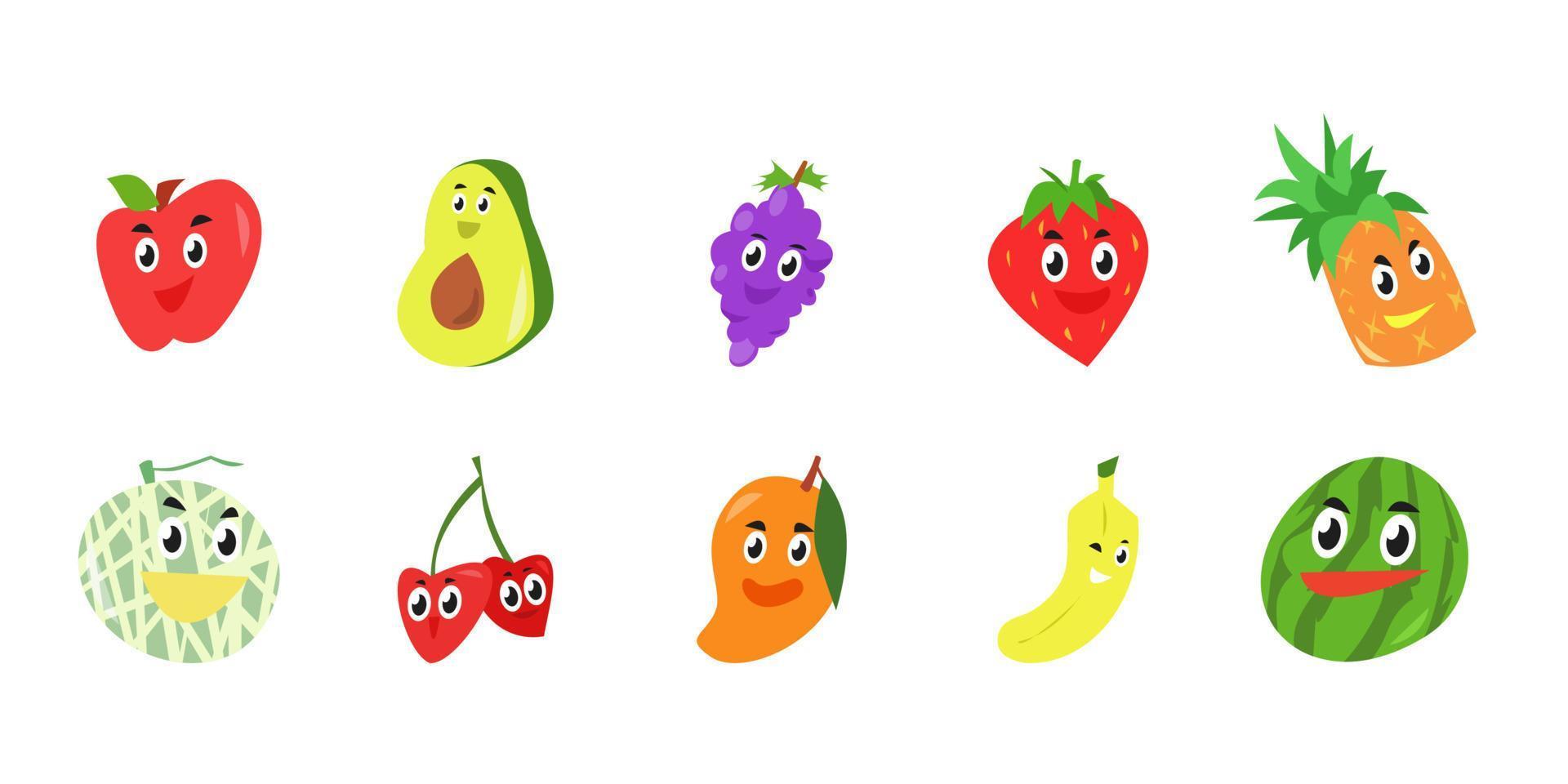This image features two rows of ten different animated cartoon fruits, each with expressive faces and big googly eyes, perfect for children's products or books. The top row showcases, from left to right, a red apple, a green avocado with a light green inside and brown pit, a cluster of grapes, a strawberry, and a pineapple, all vividly colored with simple, flat shades. The bottom row features a green melon with white stripes, two cherries with stems, an oddly-shaped orange whose form juts out slightly to the left below the mouth, a smiling banana, and a round watermelon. The fruits are all depicted as cheerful characters, adding a playful and friendly touch to their appearance.